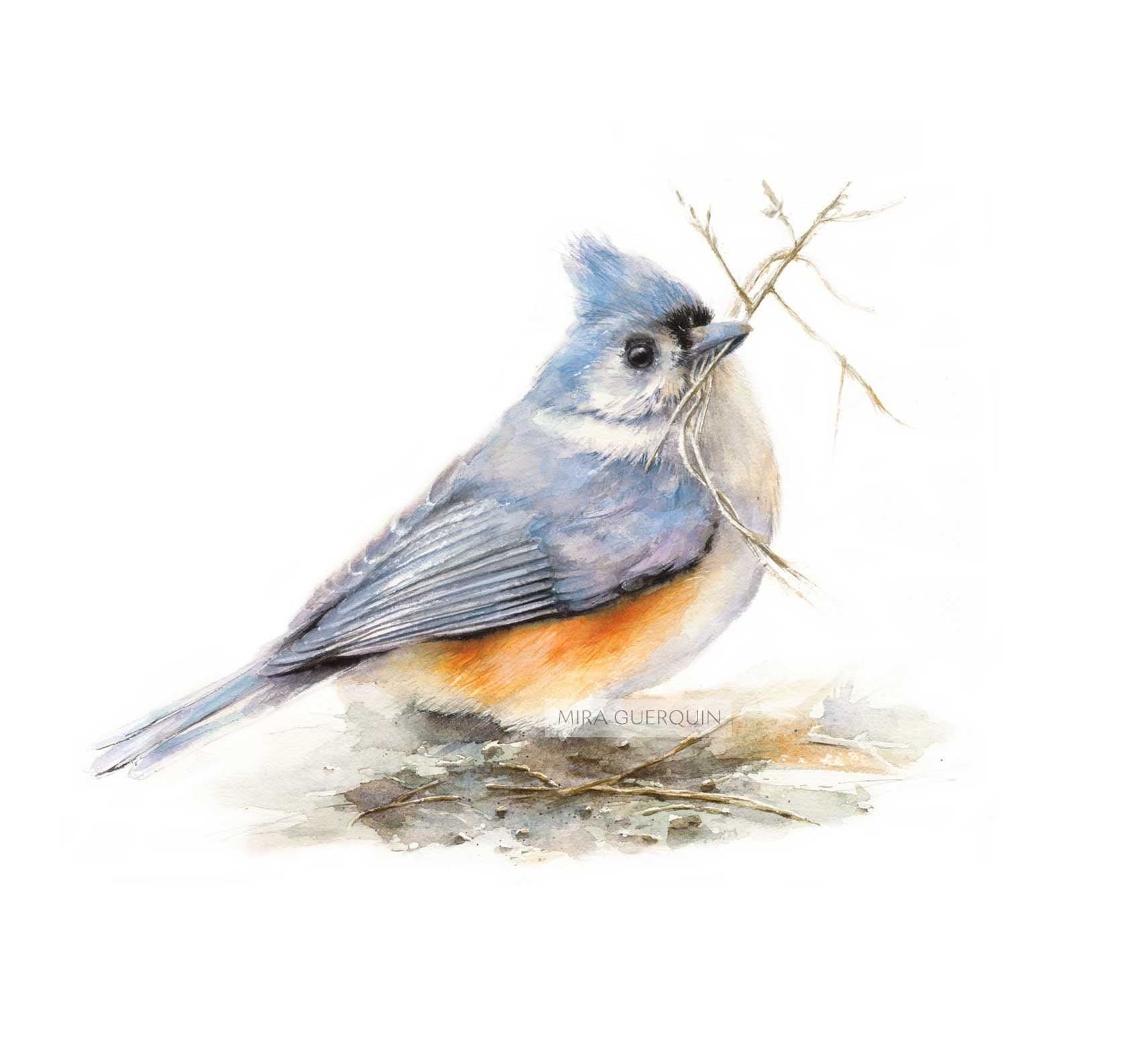This detailed watercolor painting by Mira Gherkin captures a small, plump blue bird, likely a blue jay, standing on a ground that fades out, possibly dirt and pine needles. Positioned in the center of the frame, the bird is portrayed in a side profile facing to the viewer's right, with its head slightly tilted towards the viewer. The bird's upper half is a light blue shade, featuring a distinctive triangle-shaped fluffed crest on its head. Its beak, also blue, is encircled with black at the base. Intricate details are present around its eye, including a white shading both around and below the eye, contrasted by the dark eye itself. The bird's white belly extends all the way down to its feet, with a hint of orange or light tan under its wings, transitioning to a light brownish color that extends to its blue tail which is pointed outward. Notably, the bird holds a small twig or piece of grass in its beak, suggesting it might be in the process of building a nest.